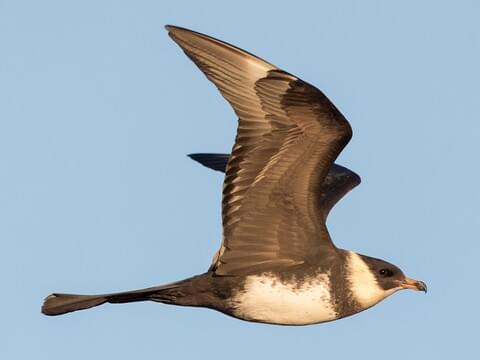This detailed photographic close-up captures a pigeon in mid-flight against a light blue sky. The pigeon’s wings are folded upward, showcasing its elongated, pointed feathers that display a blend of brown with white accents. The bird's body is straight with a narrow, rounded tail flaring out slightly at the end. Its belly is white with a distinct brown accent, while a white ring encircles its brown head, which features a striking black eye. The pigeon’s orange beak adds a vibrant contrast. Despite the uniform backdrop, the sunlight highlights the intricate details of the bird's feathers, emphasizing its purposeful flight across the serene sky.